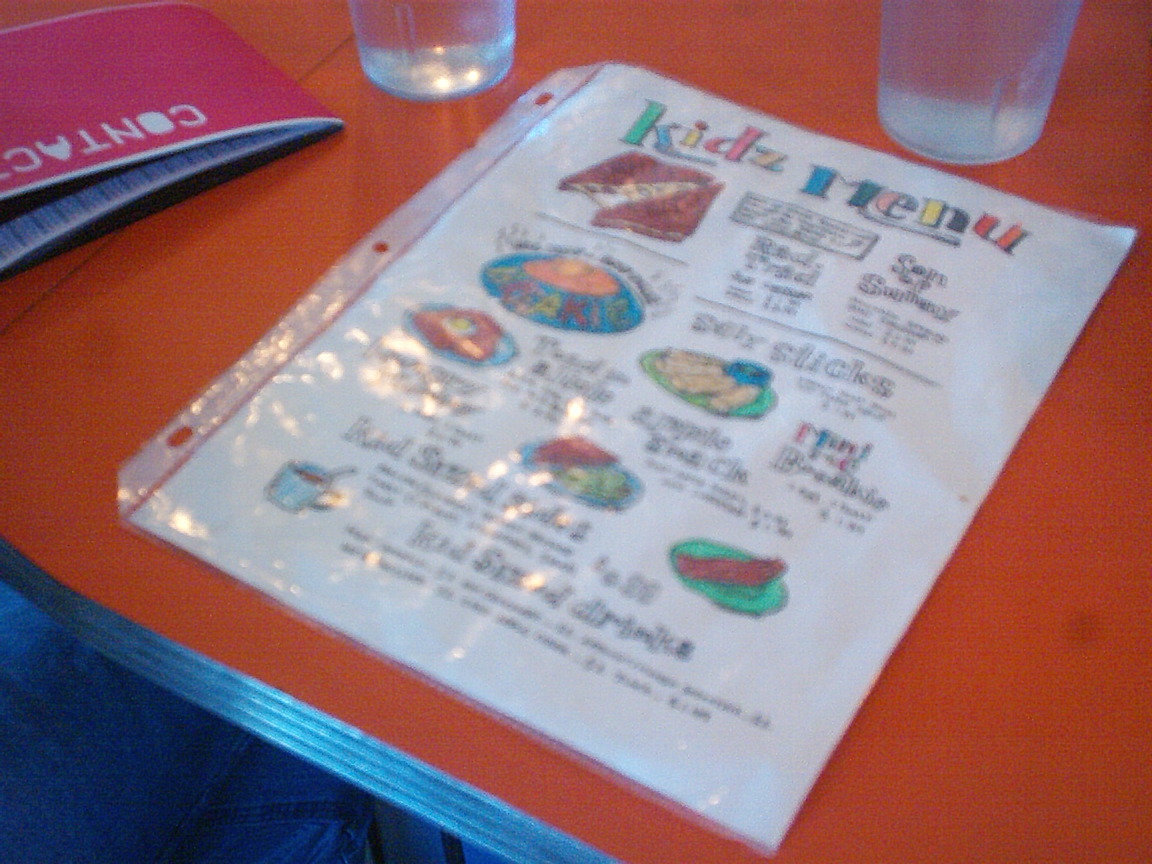This photograph, though blurred and poorly lit, captures the ambiance of a cozy restaurant or diner. The primary illumination comes from overhead lights, casting a warm glow on the scene. The brightly colored, laminate-surfaced table, with its distinctive stainless steel edge marked by a four-line grooved texture, dominates the image. A dark indigo area in the bottom left corner suggests either a person's trousers or the shadow beneath the table.

The tabletop is a vibrant orange, featuring what appears to be a seam or joint at the top left corner, possibly from the meeting of two tables. On the table are two plastic cups, one situated just left of center at the top and the other in the top right corner. The focal point of the photo is an A4-sized kids' menu encased in a protective plastic sleeve, displaying the words "Kids' Menu" in a lively, colorful font. The menu is adorned with whimsical drawings of various foods, vividly illustrated in playful hues. Additionally, in the top left corner, there is a booklet labeled "Contact," which seems to have lined pages, hinting at a restaurant checklist or guestbook. The photograph, despite its imperfections, encapsulates the cheerful and informal atmosphere typical of family-friendly dining establishments.